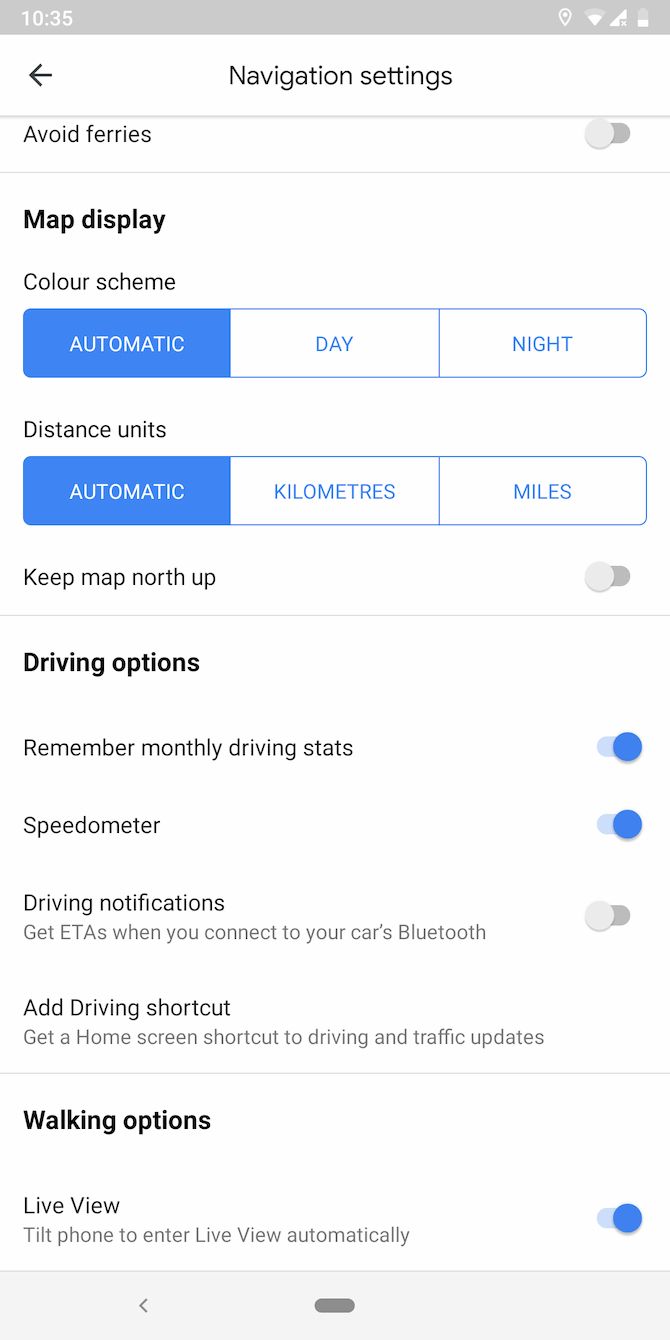The image depicts a screenshot of a website on a smartphone. Across the top, there's a gray banner. On the left side of this banner, it displays the current time in white text: "10:35." On the right side of the banner, various icons indicate the device’s status, including location, battery life, cell signal strength, and Wi-Fi signal strength.

The main content area of the screen features a white background. At the top left, there's a left-facing arrow. Centered at the top is the heading "Navigation Settings" in bold, with a capital "N." Below this heading, a horizontal line divides the screen.

The first settings option reads "Avoid ferries," which is currently turned off. Following this, the section titled "Map Display" in bold print with a capital "M" appears. Under the "Map Display" heading, there's an option for "Color screen" set to "Automatic," displayed in blue with white text. Alternative options, "Day" and "Night," are shown with white backgrounds and blue text.

The next settings group is "Distance units." The default "Automatic" option is highlighted in blue with white text, while the alternatives "Kilometers" and "Miles" are presented with white backgrounds and blue text.

Further down, the screen shows "Keep map north up," which is turned off. Beneath this, the "Driving options" section is boldly labeled with a capital "D." The settings within this section include "Remember monthly driving stats," which is turned on; "Speedometer," also turned on; and "Driving notifications," which is turned off. There's also an option to "Add driving shortcut."

Finally, the "Walking options" section follows, highlighted in bold print. The "Live view" setting in this section is turned on.